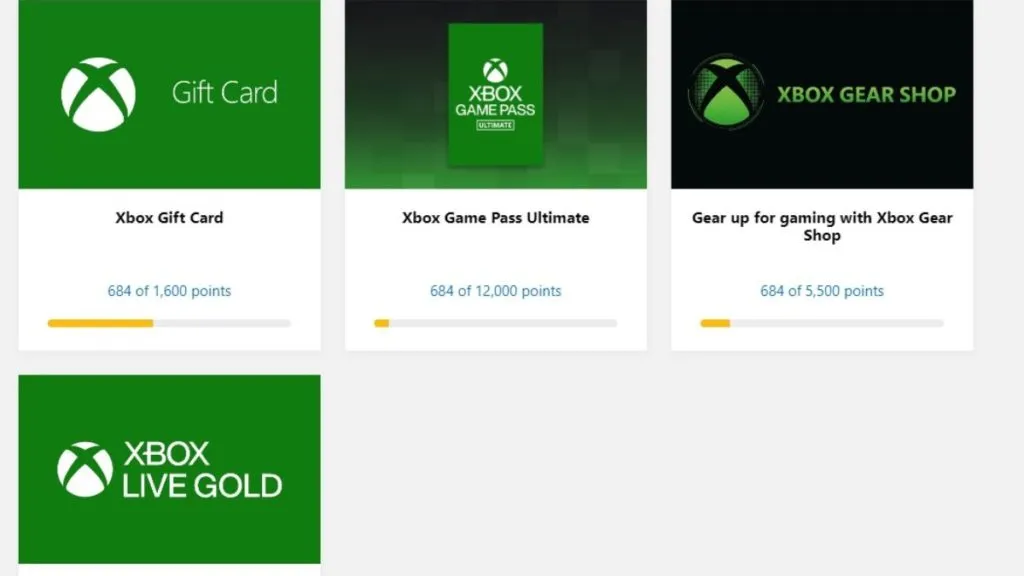This image is a promotional screenshot for Xbox Live Gold. The vibrant color scheme predominantly features green with white lettering, and sections of black with white lettering in the upper right. The window is divided into four distinct panels, each providing information on different aspects of the Xbox Live offerings.

1. **Gift Card Panel (Upper Left):**
   - **Background:** Green with the Xbox emblem prominently displayed.
   - **Text:** "Gift Card" is written in white letters.
   - **Details:** In the white section below, it says "Xbox Gift Card" followed by "684 of 1600 points" in blue letters. A yellow status bar indicates about 40% completion of the required points.

2. **Game Pass Panel (Upper Middle):**
   - **Background:** A combination of black and green with the green Xbox logo.
   - **Text:** "Xbox Game Pass" is written with a clickable button underneath.
   - **Details:** The white section below reads "Xbox Game Pass Ultimate" with "684 of 12,000 points" in blue letters. A status bar, less than 10% complete, displays progress.

3. **Gear Shop Panel (Upper Right):**
   - **Background:** Black with the Xbox logo on a black background enveloped by green accents.
   - **Text:** Reads "Xbox Gear Shop".
   - **Details:** The white section below states "Gear Up for Gaming with Xbox Gear Shop" and "684 of 5,500 points". The completion bar shows the progress to be slightly over 10%.

4. **Xbox Live Gold Panel (Bottom Left):**
   - **Background:** Green featuring the Xbox logo.
   - **Text:** "Xbox Live Gold" is written in white letters.

This detailed layout emphasizes different reward facets of the Xbox ecosystem, providing gamers with clear progress indicators for each category.